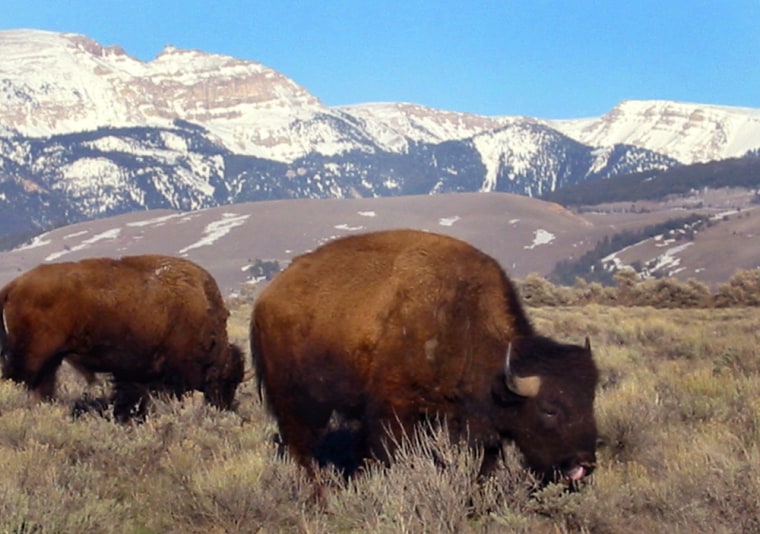In the forefront of the image, there is a flat expanse of light green grass dotted with patches of brown shrubbery. Two buffalo, or bison, stand out prominently against this pale background. The one on the left is positioned slightly towards the center, head down, grazing, with its full body visible except for the tail, which is cut off on the left edge. This bison is dark brown across its body, and its head is a darker shade of brown, with two small horns peeking out. To the right, the second bison faces the back, its round, light brown face is visible with its rear to the left of the picture. Both animals appear to be feeding on the sparse brown brush.

Behind the bison, a row of light green trees marks the transition from the flat foreground to the rolling hills and low plains in the middle ground which are dotted with patches of snow. Beyond this, an imposing mountain range rises dramatically, its peaks capped with snow. The mountains below the snowy caps range in color from dark green to brown, indicating a mix of vegetation and rocky terrain. Above this majestic landscape, a strip of light blue sky tops the image, providing a serene backdrop to the scene.